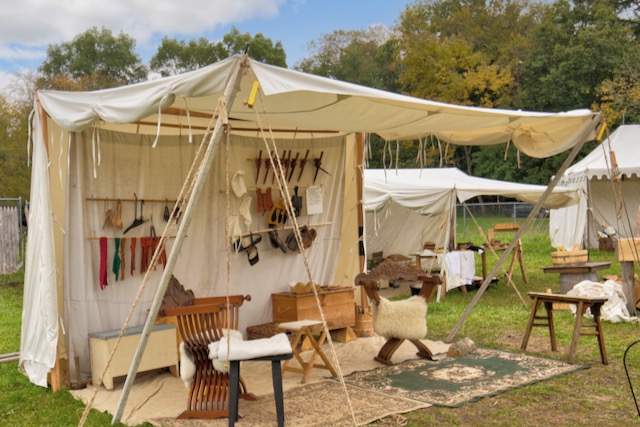This is a detailed color photograph, taken in landscape orientation, of a historical reenactment setup resembling a Civil War era medical camp. At the forefront is an outdoor tent with a white canvas canopy. The tent is open and supported by silver-colored angled rods and secured with ropes. The canopy hangs over a series of oriental-style, mismatched area rugs placed directly on the grass. 

Underneath the canopy, there is a central brown table covered with white cloth. To the left side, there's a seat with a white cushion, while on the right, a bench has a white sheepskin rug draped over it. The back wall of the tent, made of white canvas, hosts several hanging objects arranged in rows, including what appear to be wooden daggers and a slingshot. Below these items on the left side is a white chest with a blue top, and on the right, a wood-toned chest.

Surrounding the main tent are other similar white canvas tents, suggesting a larger encampment. Some equipment, made of stone and wood, is scattered outside. The entire scene is set in a grassy field bordered by dark green trees, partially enclosed by a chain-link fence in the background, indicating it takes place in some sort of park. The photograph employs photographic representationalism realism, capturing the detailed and historically styled outdoor vendor market.